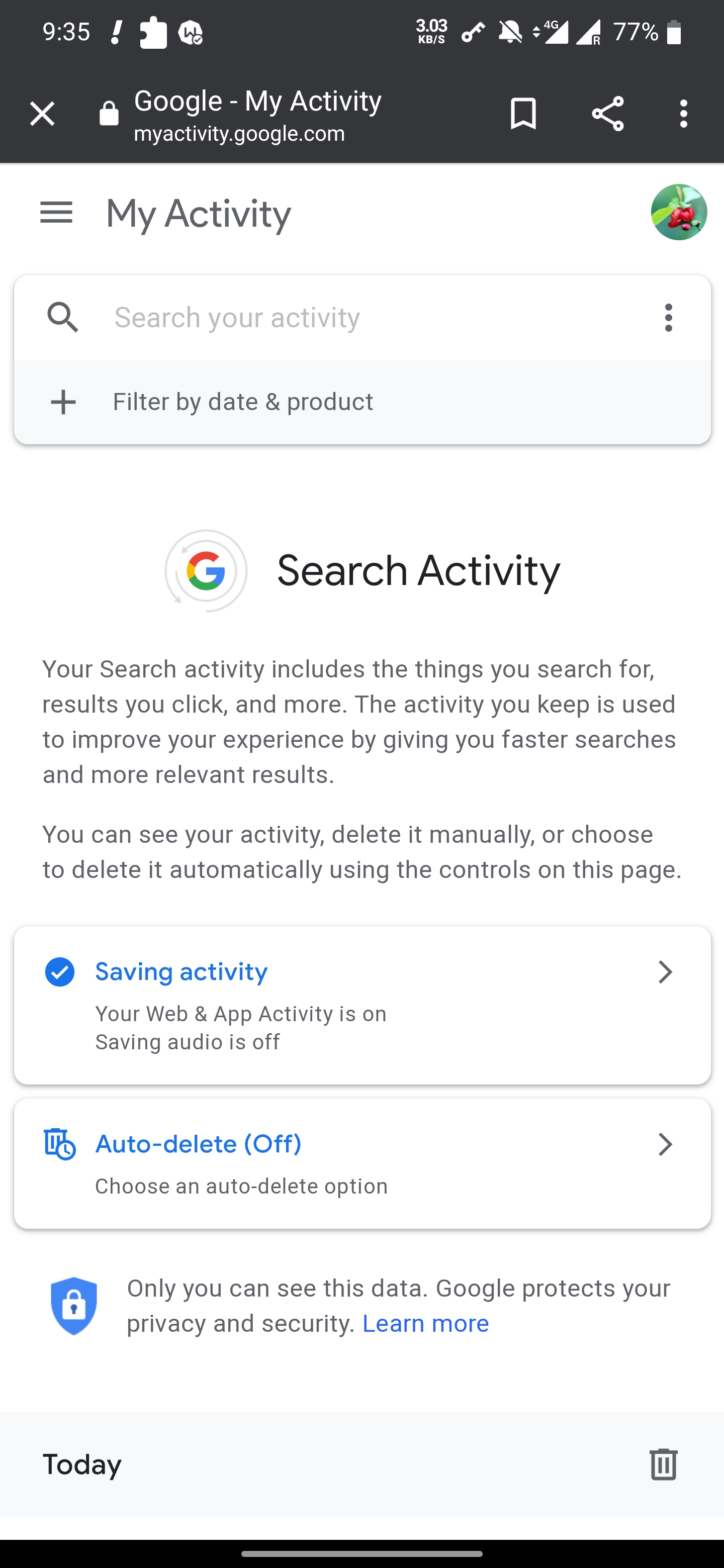This screenshot from a mobile phone captures a detailed view of a specific app screen. The top inch of the screen features a nearly black border. This area includes, from left to right, the time, a pin icon, a puzzle piece icon, and a circle with an indistinguishable letter. Moving further right, the icons represent a battery indicator showing 77%, followed by two full Wi-Fi signal bars. Additionally, there is a locked key icon and the time displayed as 3:03 PM.

Beneath this dark border, the top-left corner features a white "X" and a white lock icon. Prominently displayed are the words "Google - My Activity" in large, white letters, followed by the URL "myactivity.google.com." The same row contains a bookmark icon, a share icon, and a vertical ellipsis (three dots stacked).

The main content area of the screenshot has a white background. In the top-left corner, three horizontal black lines (a hamburger menu) are present. To the right, large text reads "My Activity," with a profile picture further to the right. The profile picture features two stick cherries on a green background. Beneath this, a search bar with a black magnifying glass icon and the text "Search your activity" is displayed. Adjacent to this, there is a "Filtered by date & product" option with a plus sign.

Below this section, there's the classic Google "G" in a white circle, next to the text "Search activity." Further down, two paragraphs of information are present, accompanied by two tabs spanning across the screen. The first tab titled "Saving activity" is highlighted in blue and displays a couple of lines underneath it, indicating "Auto-delete off."

An icon of a blue shield with a white lock appears next to some informational text. A light gray border about an inch thick encloses this section of the content. On the left, it states "Today," while on the right side, there is a trash icon.

Finally, a thin black border outlines the bottom of the screen.